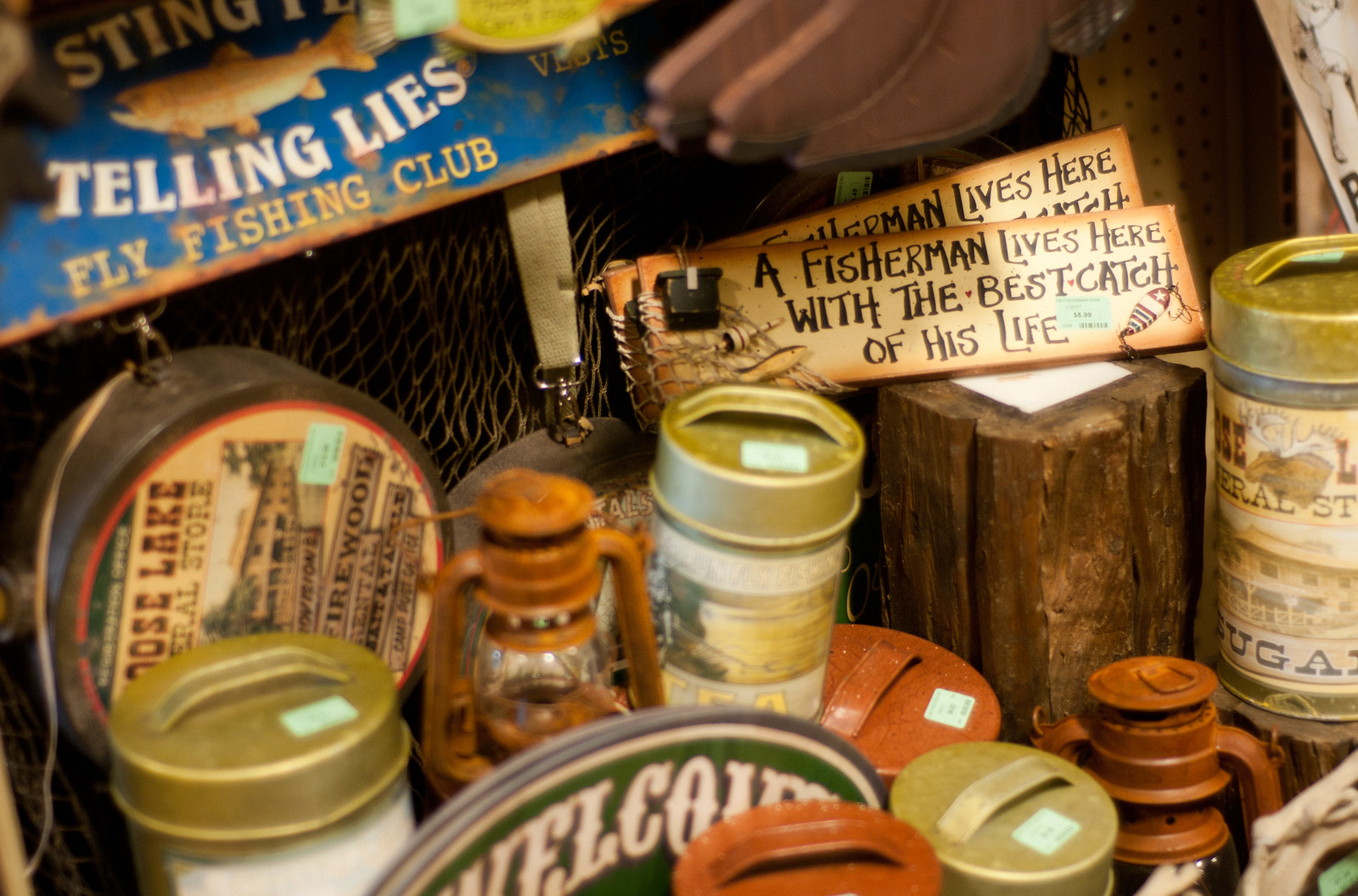The photograph depicts a detailed and eclectic assortment of items, likely taken in an antique or thrift store, or possibly a well-decorated fisherman's shack. Prominently displayed against a green backdrop is a partially visible sign with the word "STING," accompanied by an illustration of a fish, likely a bass or salmon, with the phrase "telling lies" underneath, part of a "fly fishing club" sign. Below this, netting hangs down, and to the right, a bunch of bananas dangles beside a sign which declares, "A fisherman lives here with the best catch of his life," adorned with a fishing lure symbol and a plastic bucket attached to the upper left corner. A duplicate of this sign is seen nearby. In the foreground, an old red metallic oil lantern with side handles is visible, along with various tin containers each topped with lid handles. Additional items include green-capped canteens, an oval "welcome" sign in white letters, an old sugar container with a gold lid, and miscellaneous knickknacks like wooden stumps and doodads, hinting at a collection of cherished, vintage objects. Some items have price stickers, reinforcing the notion of an antique or thrift store setting.